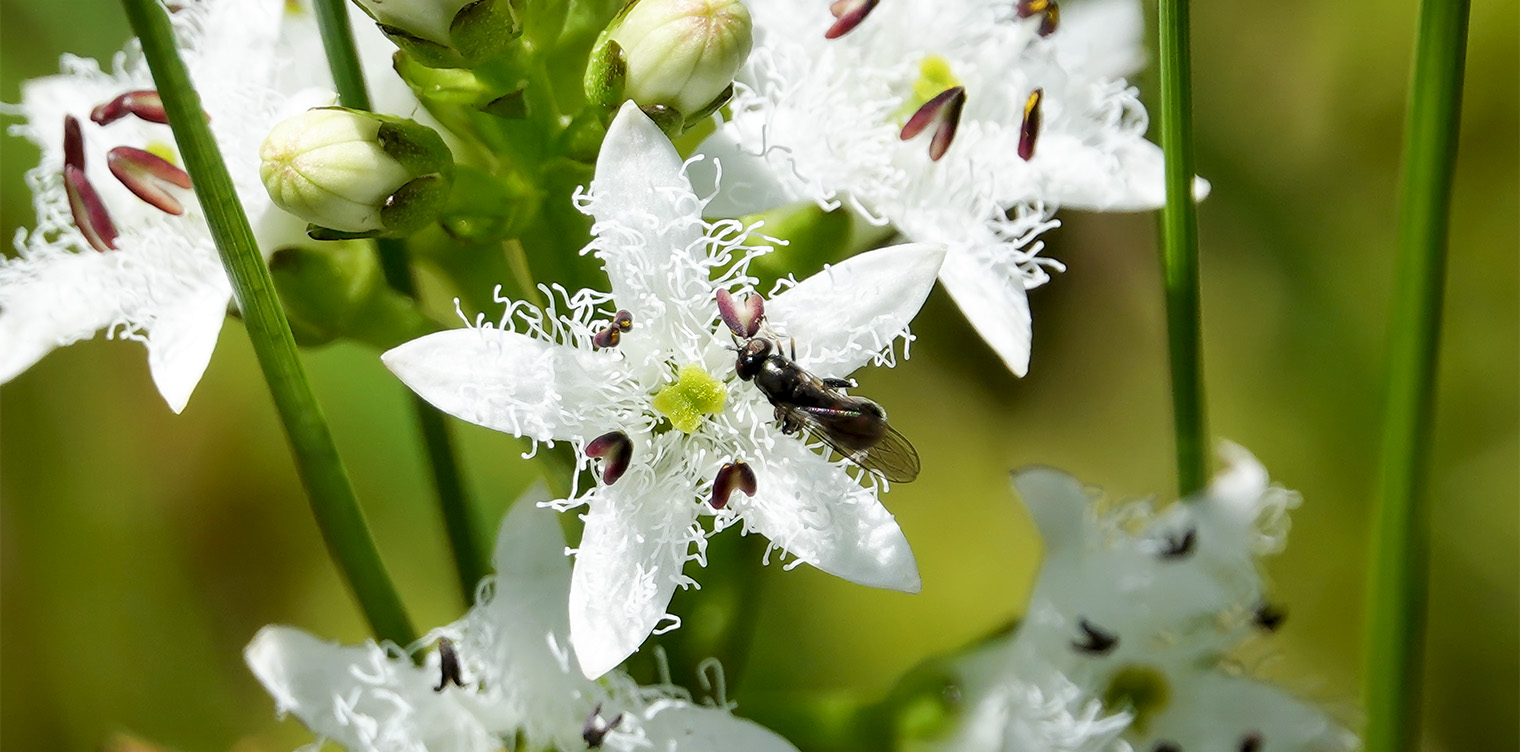This is a close-up, rectangular photograph roughly twice as wide as it is tall, capturing a cluster of white, star-shaped flowers with five petals each. The central flower, prominently featured, is bright white with a vivid yellow center and delicate, fuzzy white filaments extending from its petals. A black insect, possibly a wasp, with large wings, is perched on the right side of this focal flower. The background is muted and out of focus, creating a contrast that emphasizes the sharp detail of the central flower. Visible stems weave through the scene and behind the main flower, there are at least six other similar white flowers along with a couple of unopened buds. Although the background colors blend softly in faded greens and oranges, they enhance the vibrant whiteness of the flowers in the foreground.